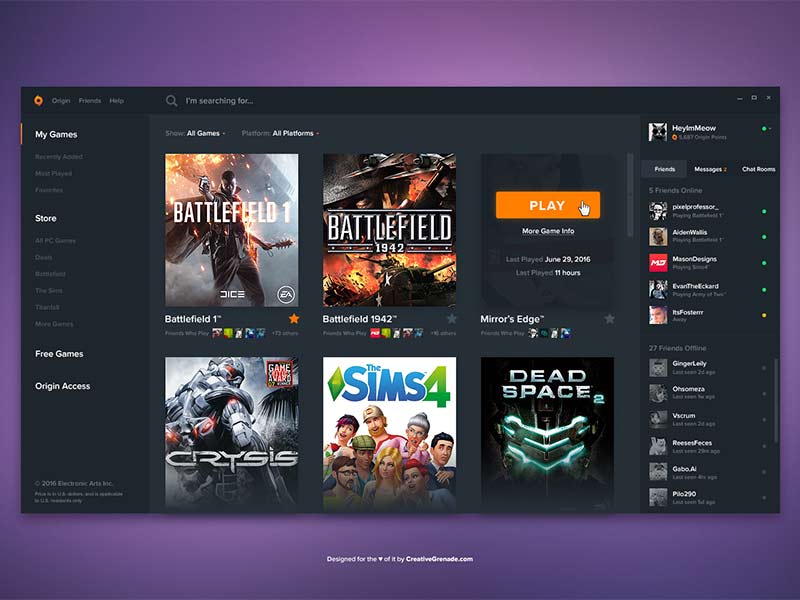The screenshot depicts a webpage dedicated to video games, framed by a striking purple square border. The screenshot is relatively small, making some of the text hard to read. The website's background is a deep dark gray, contributing to the overall moody aesthetic of the page.

Dominating the center of the screenshot are images representing five different video games. From left to right, the first image is for "Battlefield 1." It features a depiction of a warrior with the game title written in white font. Next to it is an illustration for "Battlefield 1942," showcasing a tank amid red, orange, and yellow explosions at the bottom.

On the bottom left is a cover for the game "Crysis." The title, spelled out in white letters, hovers above a gray drawing of what appears to be a monstrous figure. In the center lies "The Sims 4," with "Sims" in turquoise-blue font and the number "4" in green. This graphic includes well-rendered character drawings.

The final game on the right is titled "Deep Space," set against a black background with the title in white font. The accompanying image is ambiguous, possibly depicting a ship of some kind.

Flanking the center content are sidebars on both the left and right, also in dark gray. The right sidebar contains tiny, hard-to-decipher images of games, while the left sidebar lists various sections: "My Games" in a prominent headline, followed by "Store," "Free Games," and "Origin Access," written in white against the gray background.